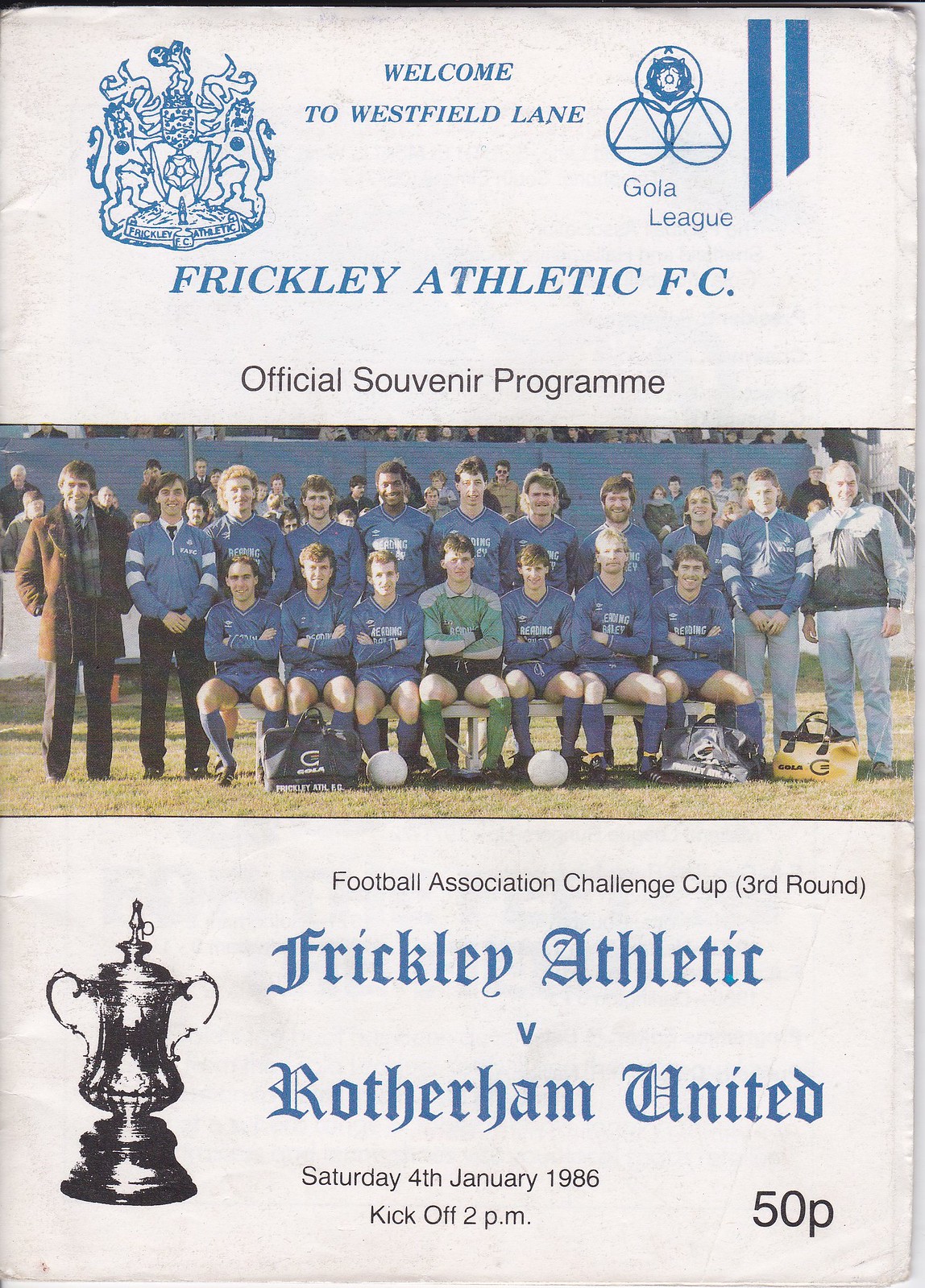This image is a scan of an old, white program or pamphlet cover from Frickley Athletic FC, specifically their Official Souvenir Program. The cover commemorates the Football Association Challenge Cup 3rd Round match between Frickley Athletic and Rotherham United, scheduled for Saturday, January 4th, 1986, with a kickoff at 2 p.m., and priced at 50p. 

At the top, the words "Welcome to Westfield Lane GOLA League" can be seen, with the Frickley Athletic FC insignia prominently displayed beneath it—a crest featuring two lions standing upright with their paws on a trophy. Flanking the insignia are crests; on the upper left is one for Frickley Athletic with a crown-like design, and on the upper right is the GOLA League insignia, consisting of three circles forming a triangle, both rendered in blue text.

The main image is a black-and-white photograph of the team positioned centrally on the cover. The team is shown posing for the photo; the front row of players is seated, dressed in blue, except for the central member in green. The back row stands behind them, accompanied by coaches positioned on the left and right edges of the group. Adding to the nostalgic atmosphere, another black-and-white photo—a trophy—sits to the left of the team photo. The setting appears to be outdoors on a soccer field, in daylight.